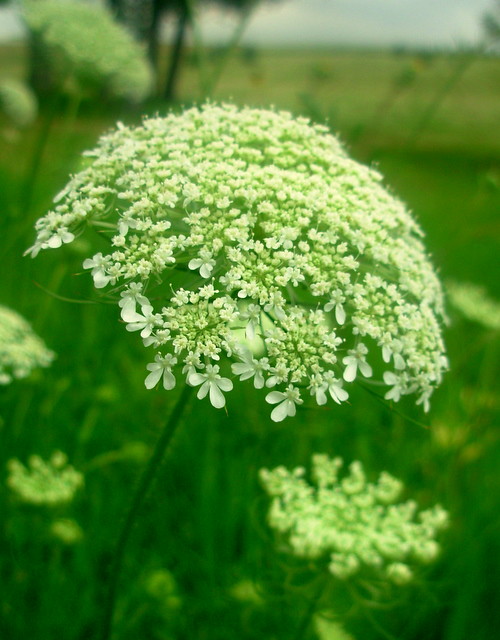In the foreground of this high-definition image, a single green stem supports a large, white wildflower with numerous delicate petals forming a canopy-like structure, suggesting it is in full bloom. The photograph reveals multiple smaller, similar flowers surrounding the central bloom, all extending their petals skyward. The background is a lush, green blur, indicating a field or garden filled with wildflowers, grass, and a hint of a tree trunk. The scene is captured under a cloudy, gray sky, adding a somber tone as the flowers seem to lean rightward, possibly under the influence of a pre-storm breeze. The image, focused sharply on the central stem and flower, fades into an impressionistic blur, framing the vibrant botanical subject against the muted hints of an impending rain.